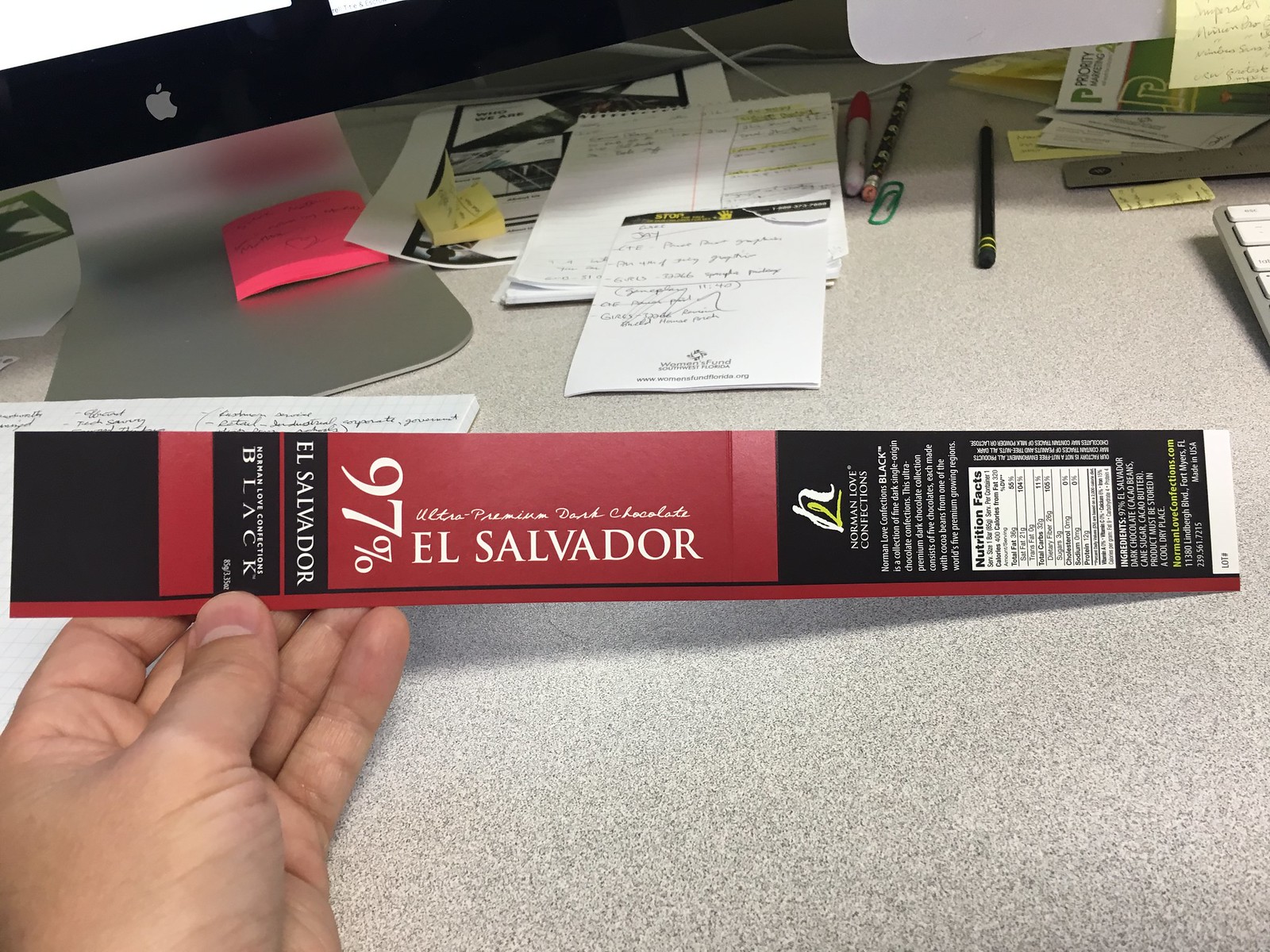In the image, a narrow, long chocolate bar is held by someone’s hand over a white and gray desk. The chocolate bar, approximately 12 to 16 inches in length and 3 to 4 inches in width, features a predominantly black and red label. The label, adorned with white text, prominently states "97% Ultra Premium Dark Chocolate, El Salvador." The front of the label is visible, as well as a section showing the nutrition information in smaller, less readable text. In the background, an office setting is apparent, with a Mac computer, stacked notepads, pens, pencils, and a distinguishable green paper clip scattered across the desk.